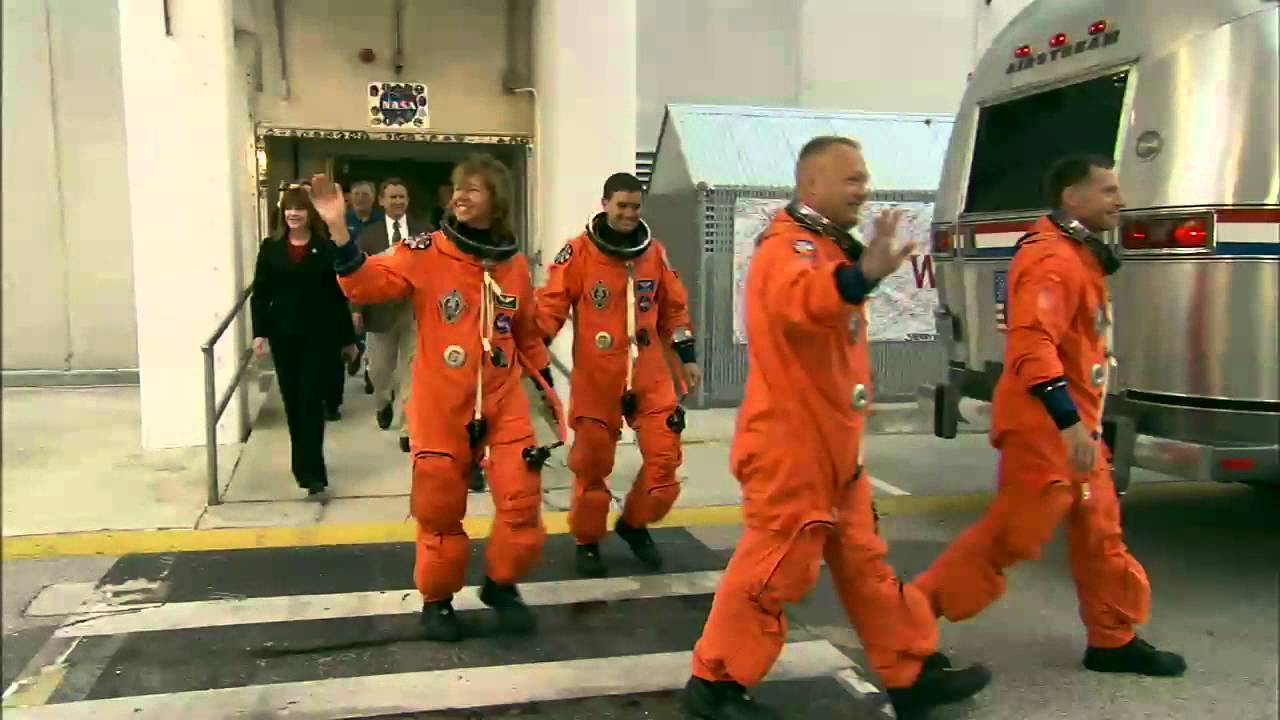In this image, there are four men dressed in solid orange outfits resembling astronaut suits, complete with blue, green, and white circular patches, and metallic elements around the neck and left side. Each is smiling. They are accompanied by a woman also in an orange space suit. Standing behind them is a woman dressed in black and a man in a brown suit, with additional people blurred in the background, all emerging from an entry or exit way. The scene appears to be set in a white parking garage, distinguished by a yellow line that transitions into a black and white crosswalk. To the right of the group, a silver Airstream vehicle is visible, marked by a red, white, and blue stripe down its middle, and a gray building with a white roof and a white banner is situated behind it.